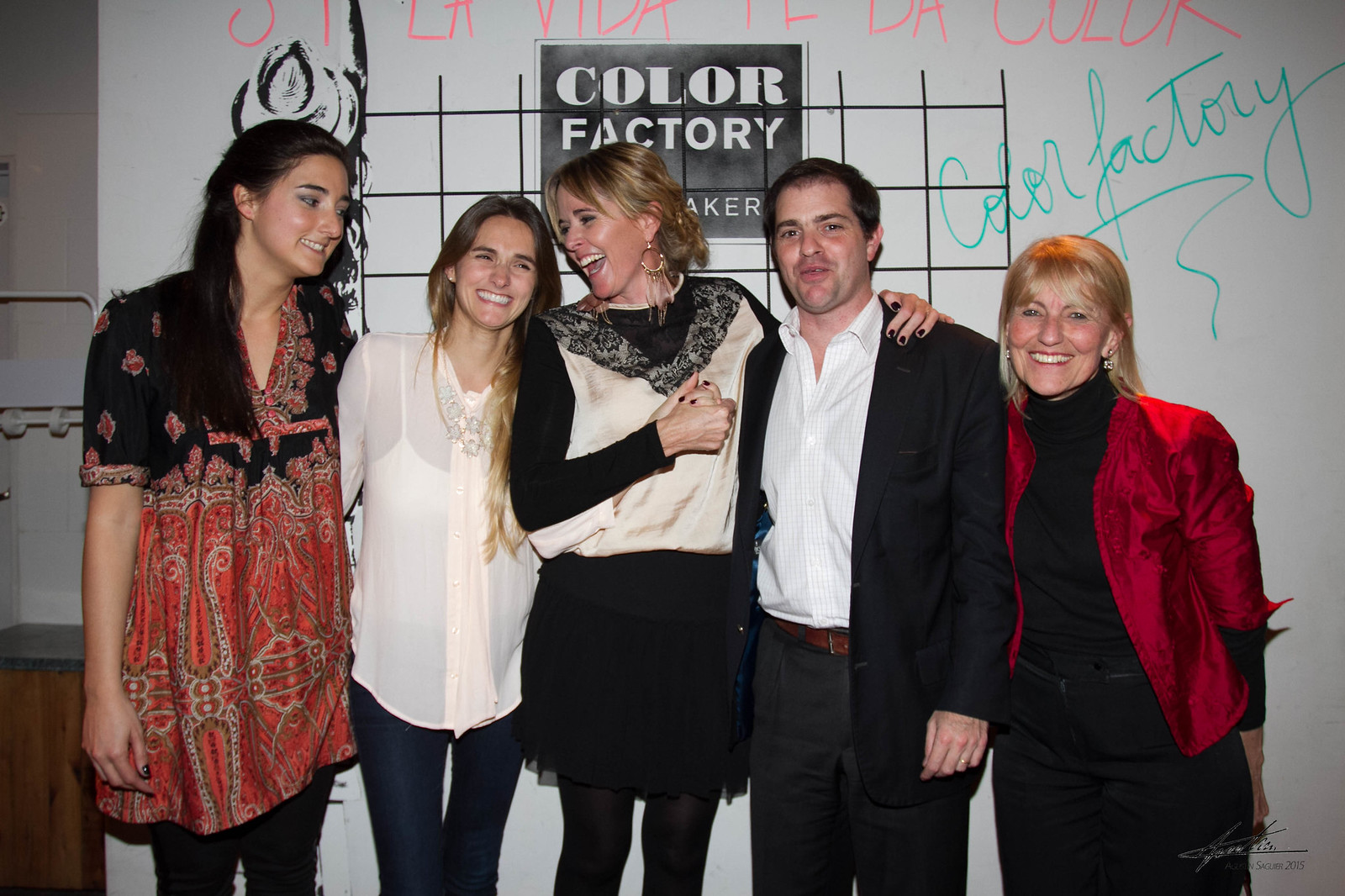This vibrant photograph features a joyful group of five young adults—four women and one man—standing in front of a whiteboard decorated with handwritten messages and signs. Central to the setting is a distinct black sign with bold white lettering that reads "Color Factory," accompanied by another script-style handwritten "Color Factory" in aqua blue and a top message in pink cursive that says "Si la vida es el color." The photo exudes a light-hearted atmosphere, possibly a party or a casual event, with all individuals dressed in a stylish blend of casual work attire and more whimsical, expressive outfits.

Starting from the left, the first woman sports a vibrant, multicolored, Indian-print top over black leggings, her long black hair cascading down her shoulders. Beside her, the next young woman is dressed in black pants and a semi-sheer white blouse over jeans, her long hair similarly flowing. The woman in the center, framed by her black frilly skirt and white bodice top with long black sleeves, smiles warmly with her arm affectionately around the gentleman. 

This gentleman, standing tall with a friendly smile, has short dark hair and dons a dark gray suit jacket paired with gray slacks, a brown belt, and a crisp white button-down shirt. Finally, the lady on the far right, shining with a big smile, has straight brown-blonde hair with bangs, and wears a striking red satin jacket over black pants and a black turtleneck shirt. The overall setting and the chemistry among the group hint at a close-knit camaraderie, capturing a moment of shared delight and color-inspired fun.